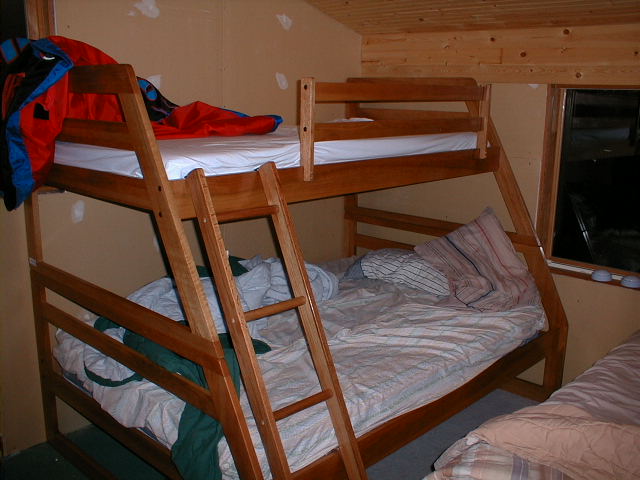The image captures a detailed scene of a children's bedroom, showcasing a dark wooden bunk bed against a light brown beige wall marred with white patches, likely indicating unfinished repairs. The top bunk, slightly smaller than the bottom, has a mattress covered with a white sheet and a loosely hanging red and blue blanket over its left railing. A wooden ladder provides access to the top bunk.

The bottom bunk features mismatched bedding: red, white, and blue striped sheets paired with a green comforter, which is piled messily near the back. No pillows are visible on either bunk. To the right, in the lower corner of the image, part of a third bed with a light pink checkered comforter suggests another sleeping area, possibly for a girl.

A medium-wood framed window without curtains is visible between the beds on the back wall, adding to the room's unfinished look. The flooring is a medium, dusty blue, adding a cool tone to the room's subdued color palette. The overall scene portrays a rustic, slightly chaotic bedroom with an unfinished and homey feel.